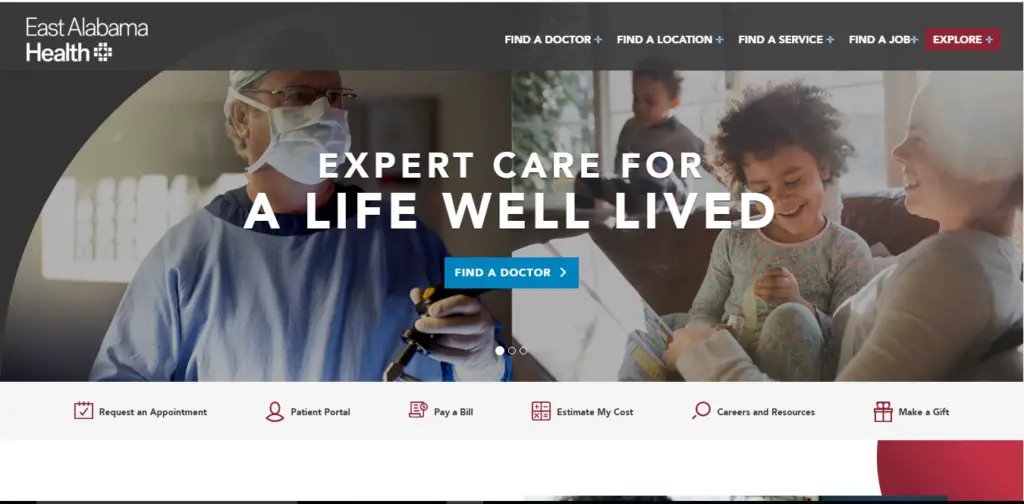The image features the East Alabama Health website. In the top left corner, the site's logo is prominently displayed. To the right of the logo, there are five navigation categories arranged horizontally: "Find a Doctor," "Find a Location," "Find a Service," "Find a Job," and a prominently highlighted "Explore" button with a red background. Below the navigation bar, the main section is divided into two parts. On the left side, there's an image of a doctor dressed in blue scrubs, wearing a white mask and glasses, and holding an object in their right hand. On the right side of the main section, there is a heartwarming scene of a mother and her two children lying on a brown couch. Centered in this section, a large text in white reads, "Expert care for a life well-lived," followed by a blue button labeled "Find a Doctor" in white letters. Beneath this, six categories are listed horizontally: "Request an Appointment," "Patient Portal," "Pay a Bill," "Eliminate My Cost," "Careers and Resources," and "Make a Gift." The overall background of the webpage is white, while the bottom right corner has a red section. The top of the page, including the top left area behind the logo, features a dark gray background.